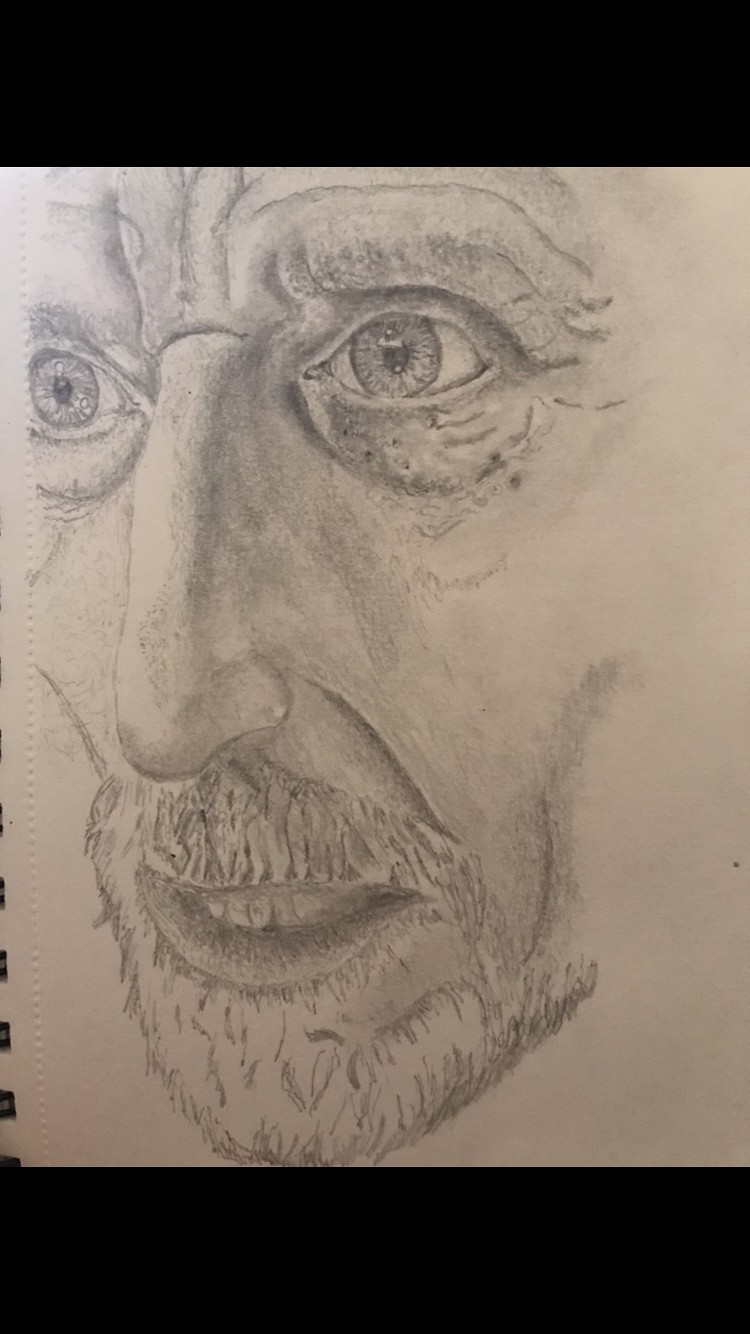The image showcases a highly detailed black and white pencil drawing of an older man’s face in a spiral-bound notebook, with the black metal spirals visible at the bottom left of the picture. The drawing is exceptionally realistic, capturing the man's expressive features with precision. His face is adorned with a neatly trimmed beard and mustache, and his eyes are wide and large, complete with carefully rendered irises. Deep creases and furrowed lines mark his forehead and the area between his brows, while additional wrinkles appear around his eyes and along his face. His nose is long and thin, and his slightly open mouth reveals some crooked teeth, indicating a look of surprise or shock. The paper's white background contrasts beautifully with the varying shades of gray, emphasizing the drawing's intricate details and the artist’s skill.